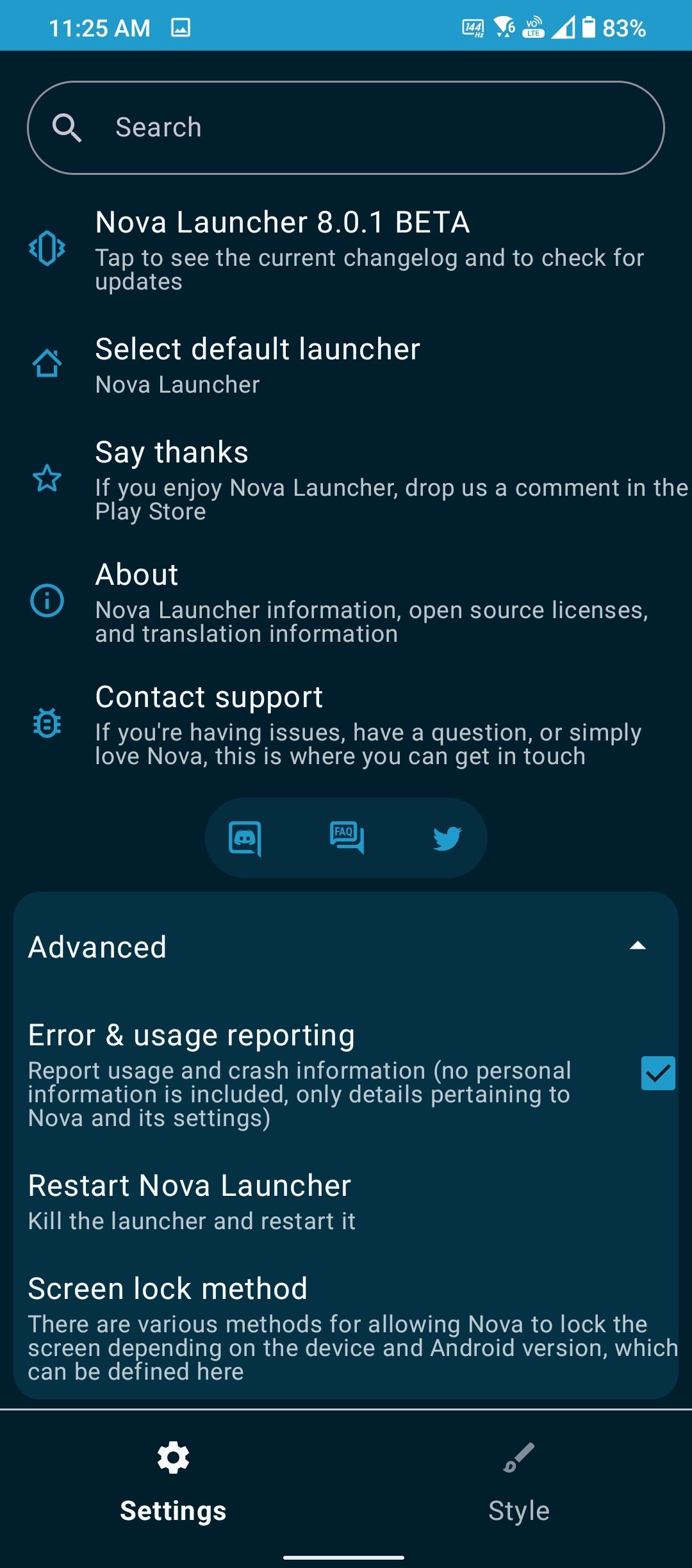Here's a detailed and refined caption for the given screenshot:

---

This smartphone screenshot, captured at 11:25 AM, showcases a device with Wi-Fi and cell reception signals, and a battery at 83% charge. The interface is centered around a Nova Launcher settings page. At the top, a search bar is positioned within a black header backdrop. Below the search bar, a list of options is presented:

1. **Nova Launcher 8.0.1 Beta**: Tap to view the current changelog and check for updates.
2. **Select Default Launcher**: Choose Nova Launcher as the default home screen launcher.
3. **Say Thanks**: If you enjoy Nova Launcher, leave a comment on the Play Store.
4. **About Nova Launcher**: Includes information, open source licenses, and translation details.
5. **Contact Support**: Reach out for support, ask questions, or provide feedback.

Below these options is a distinctive blue rectangle labeled "Advanced." This section includes:

- **Error and Usage Reporting**: Share usage and crash data, excluding personal information, related to Nova settings.
- **Restart Nova Launcher**: Terminate and restart the launcher.
- **Screen Lock Method**: Define screen locking methods based on the device and Android version.

At the bottom of the screen, there is a footer labeled "Settings and Style."

---